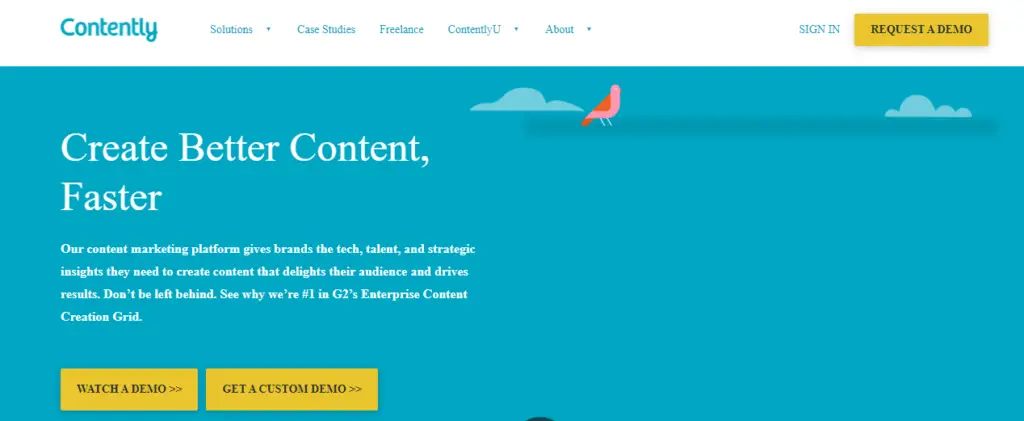The Contently website features a predominantly blue and white-themed background, with text mainly in blue, accented by white. At the very top, there is a white header where the "Contently" logo is positioned to the left. Adjacent to this logo are several menu options listed horizontally: Solutions, Case Studies, Freelance, Contently You, and About. On the far right of the header, there are options to sign in or a prominent yellow button labeled "Request a Demo."

Beneath the header lies a large rectangular blue section adorned with cloud graphics and an animated bird. On the left side of this section, the tagline "Create Better Content Faster" is prominently displayed in large letters. Below this, a smaller text elaborates: "Our content marketing platform gives brands the tech, talent, and strategic insights they need to create content that delights their audience and drives results. Don't be left behind. See why we're number one in G2's Enterprise Content Creation Grid."

At the bottom of the blue section, there are two yellow buttons: "Watch a Demo" and "Get a Custom Demo," inviting visitors to further explore the platform's capabilities.